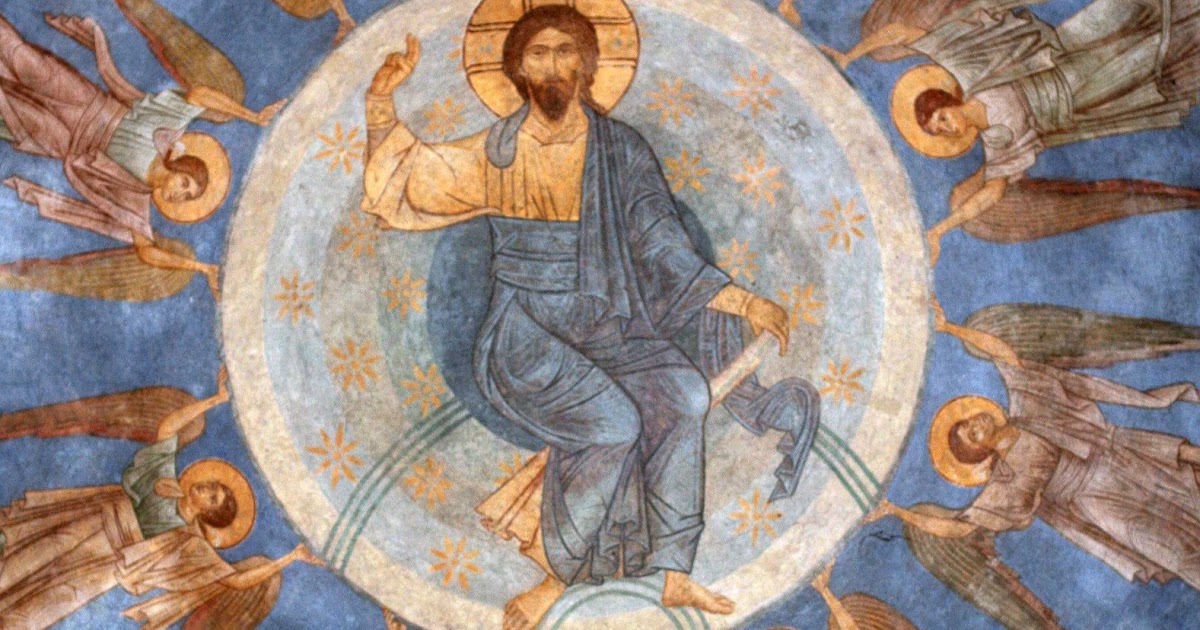The image depicts a painting of Jesus Christ, seated in the center of a large, elaborate circular design. Jesus is barefoot, with a full beard, brown hair, and a brown hat patterned like a tic-tac-toe grid. He is dressed in a white shirt and a blue robe draped over his shoulder and legs. His right arm is raised, with his pointer and middle fingers extended in a gesture resembling a peace sign, while his left hand rests on a chair. Surrounding Jesus are four angels, symmetrically positioned and seemingly lifting or supporting the circular frame around Jesus. These angels resemble each other, wearing similar yellow hats, white robes, and blue garments, with wings and circular halos around their heads. The circle itself features intricate floral patterns in shades of white, light blue, and dark blue, resembling star-like or flower-like designs. The outer parts of the circle are colored dark blue, creating a visually striking contrast that frames and accentuates the central figure of Jesus and the surrounding angels.